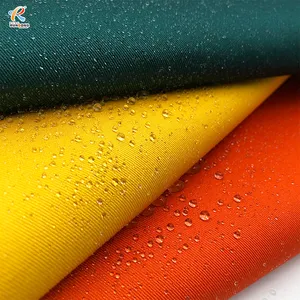The image captures three bright fabrics stacked atop one another on an unseen white surface, only partially visible in the bottom right corner. The fabrics are oriented diagonally from the lower left to the upper right, creating a layered appearance. The top fabric is a dark green, followed by a yellow fabric in the middle, and a red fabric at the bottom. Each fabric is adorned with numerous water droplets, suggesting they are waterproof or recently exposed to water. In the bottom left corner of the image is a distinct logo featuring the capital letter "R," which is divided into yellow on the left side, red on the top loop, and blue on the lower leg. The overall composition creates a vibrant and dynamic visual, emphasized by the reflective water droplets on the smooth surfaces of the fabrics.